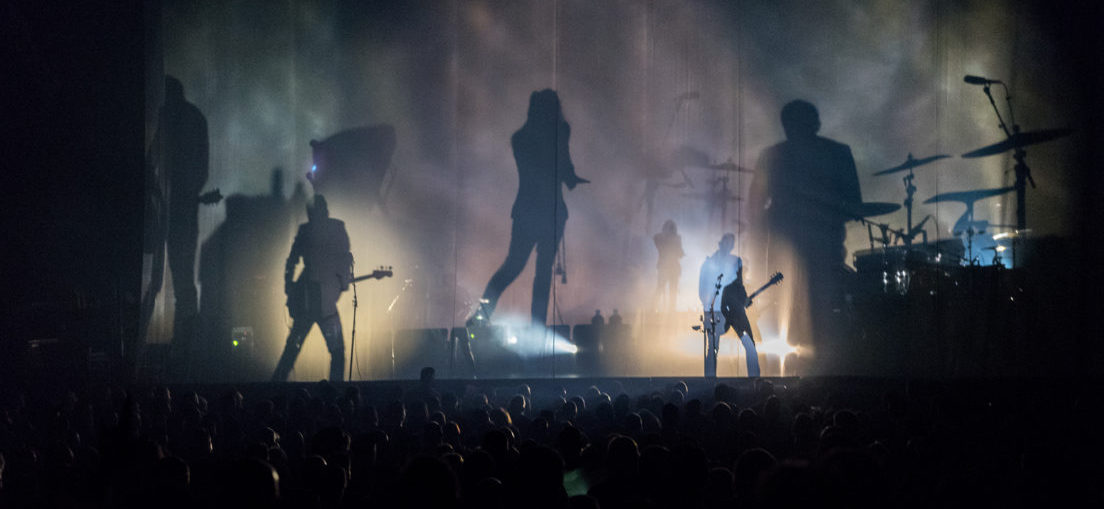This image captures the dynamic atmosphere of a dimly-lit concert from the perspective of the back of the audience. The crowd stands enraptured, their silhouettes blending into the scene's dark ambiance. Up on stage, a dramatic play of light and shadow casts the performers as larger-than-life black silhouettes. The band members, including a lead singer, two guitarists, and a drummer, are backlit in such a way that they appear as towering shadows, creating a powerful visual effect. The stage is bathed in soft, muted colors – hues of yellow, pink, and blue – but these lights only serve to deepen the shadows, giving the impression of a hazy curtain obscuring the performers. This shadowy projection either originates from behind or is carefully imposed over the band, enhancing the larger-than-life silhouette effect. The scene's mystery and grandeur are heightened by the indistinct yet energetic presence of the musicians and the audience's engaged silhouettes.